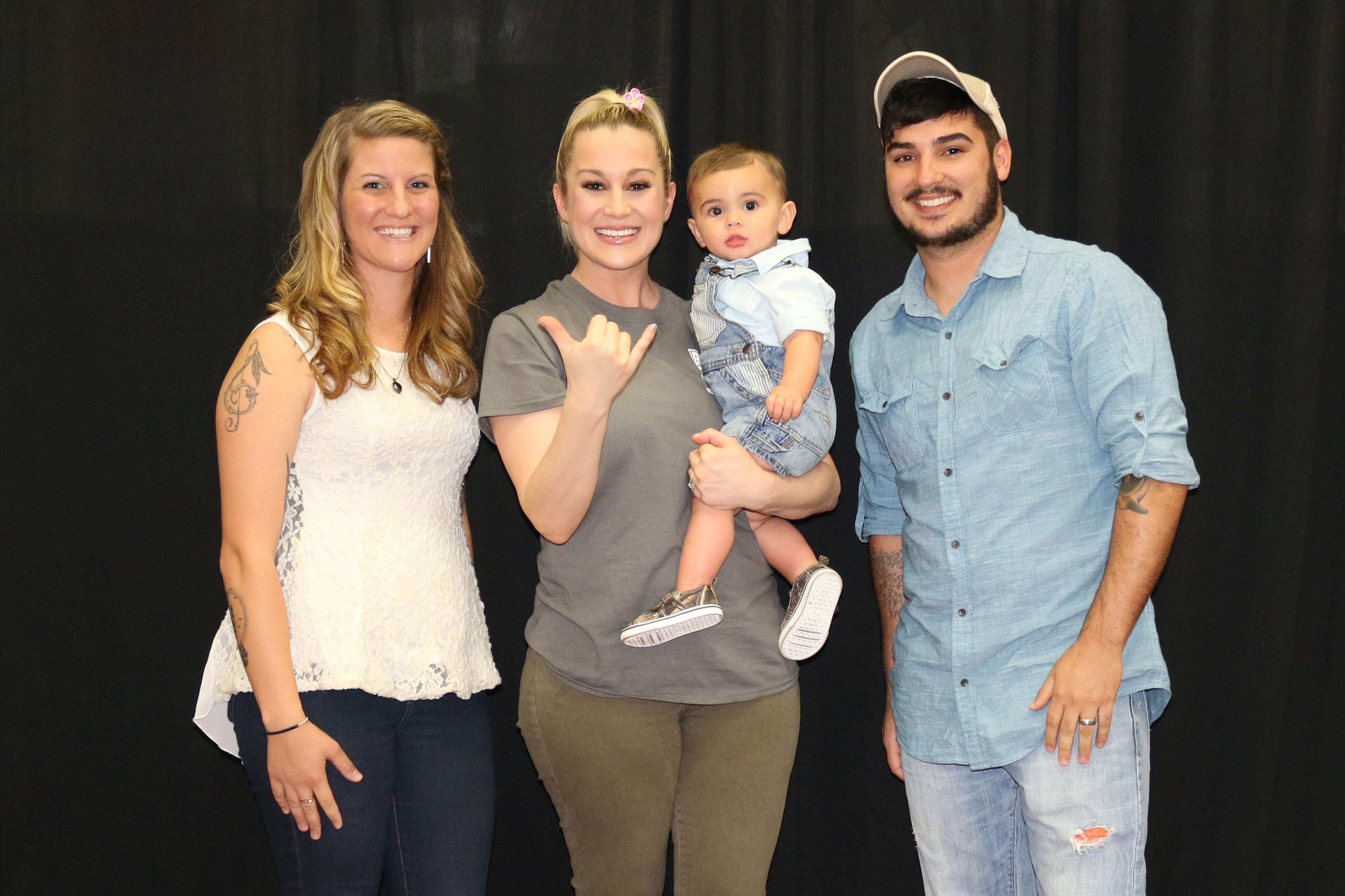In this likely professionally taken photograph, four individuals stand centered in front of a black show curtain, all smiling for the camera. On the left is a smiling blonde woman with long hair wearing a white sleeveless tank top, blue jeans, and sporting a tattoo on her right arm. To her side is another blonde woman, identified by her hair being put up, dressed in a gray t-shirt and medium tan jeans. She is holding a little baby boy clad in a white shirt, denim trousers, and camouflage sneakers, making an aloha gesture with her right hand. This woman in the gray shirt appears older and could very well be a recognizable celebrity, given the posed nature of the group. To the right, a man with dark hair, a goatee, and a white baseball cap stands wearing a light blue button-down shirt and light-colored jeans. They seem to be posing for a possible meet and greet with the central woman, whose presence suggests some level of fame, although there is no text or context confirming this. The baby looks indifferent, adding a touch of innocence to the photo.